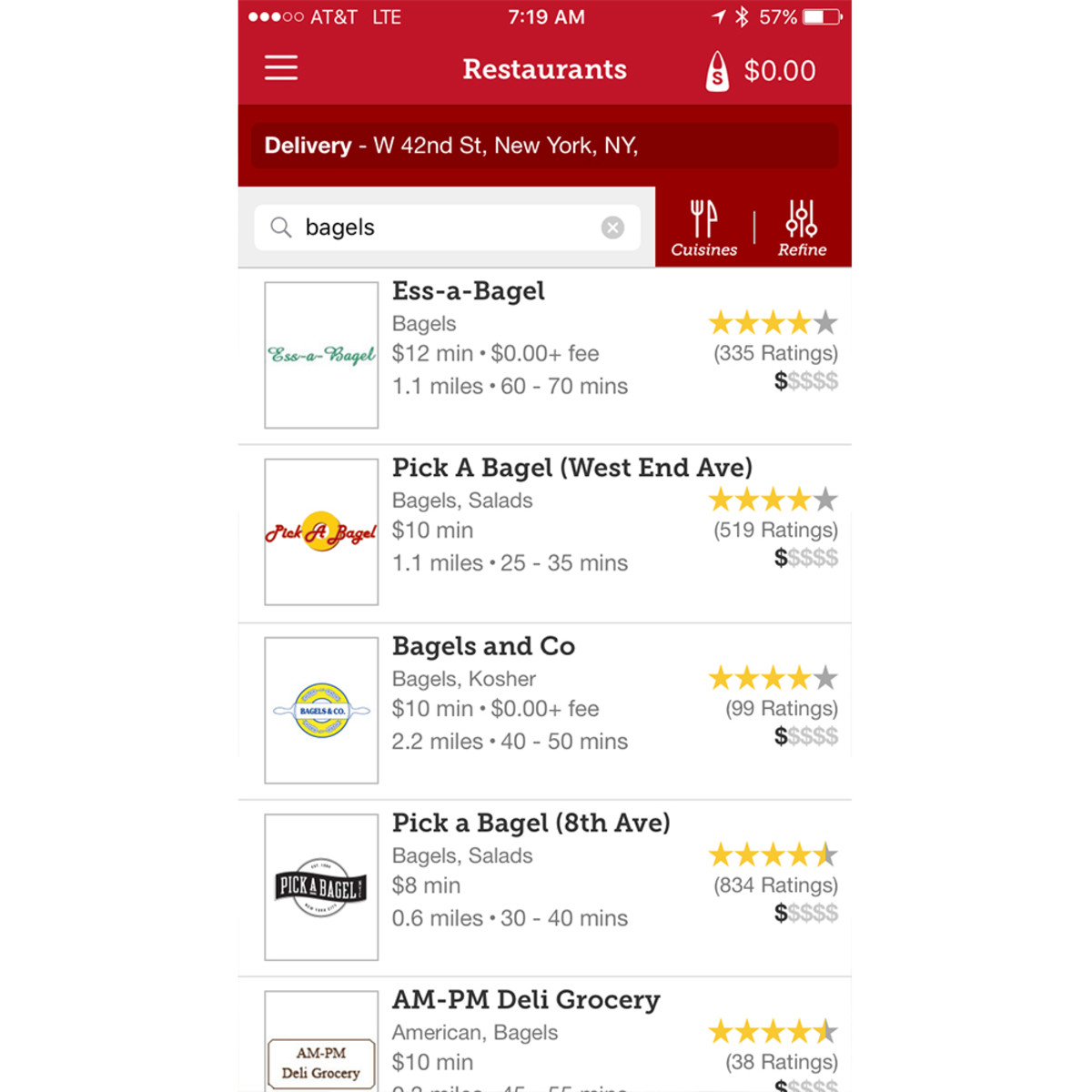In this mobile screenshot, we observe an interface highly reminiscent of a DoorDash layout, distinguished by its predominantly rose-red color scheme. The screenshot displays a search for "bagels," yielding five visible results.

At the top of the list is "S Bagel," boasting a rating of four stars out of five from 335 reviews and categorized by a single dollar sign, indicating affordability. Following is "Pick a Bagel, West End Avenue," also with a four-star rating and a single dollar sign. The third option, "Bagels and Co.," maintains the four-star rating and one dollar sign as well. 

Moving down the list, "Pick a Bagel, 8th Avenue" stands out slightly with a four and a half star rating, still maintaining a single dollar sign. Lastly, "A.M. P.M. Deli Grocery" shares this four and a half star rating and one dollar sign, signifying both quality and affordability.

To the left of each restaurant name, their corresponding logos are displayed. The interface also provides additional details, such as the types of food each establishment offers and their distance from the user's current location.